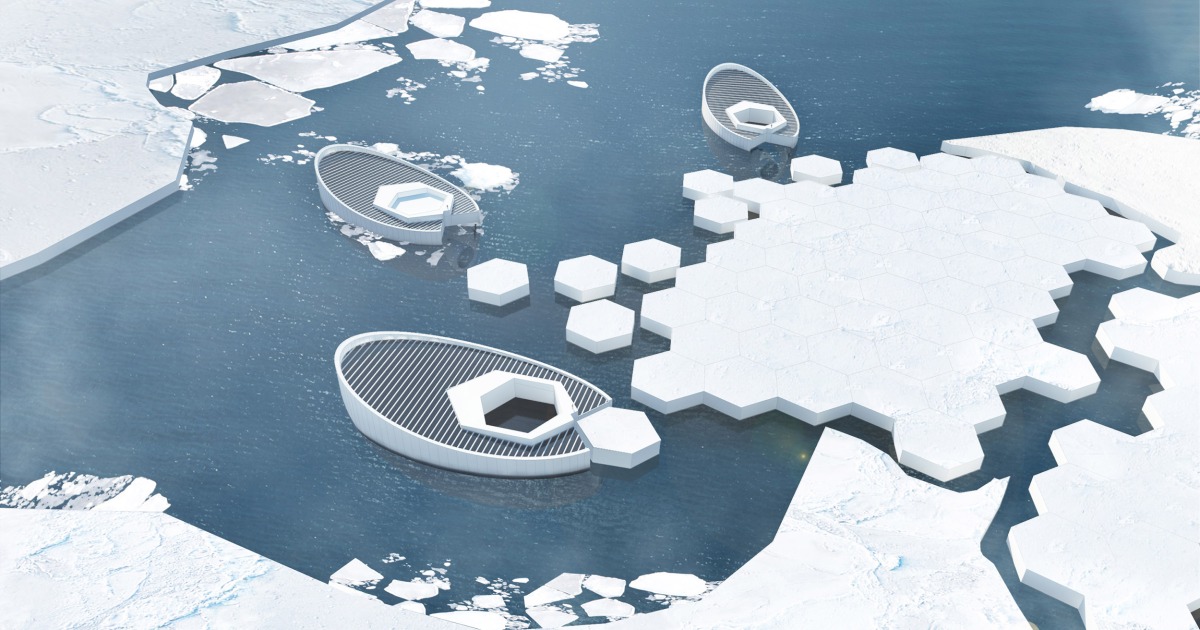This image is a highly detailed, computer-generated 3D rendering of a cold, polar-like seascape. The water is depicted in a rich, dark blue shade, and it is dotted with variously shaped icebergs. Most strikingly, a central iceberg is fragmented into perfect hexagonal pieces, resembling a meticulous, artistic design.

There are three oval-shaped vessels floating on the water, designed with vertical and horizontal gray stripes on their gray decks. A notable feature is a cutout in the center of each vessel, two of which reveal glimpses of the water beneath, while the third is obscured by a white geometric shape.

The icebergs and vessels together create a striking contrast of natural and geometric forms, generating a sense of surreal artistry. The detailed textures and absence of human presence make the scene appear realistically rendered yet otherworldly in its perfection.